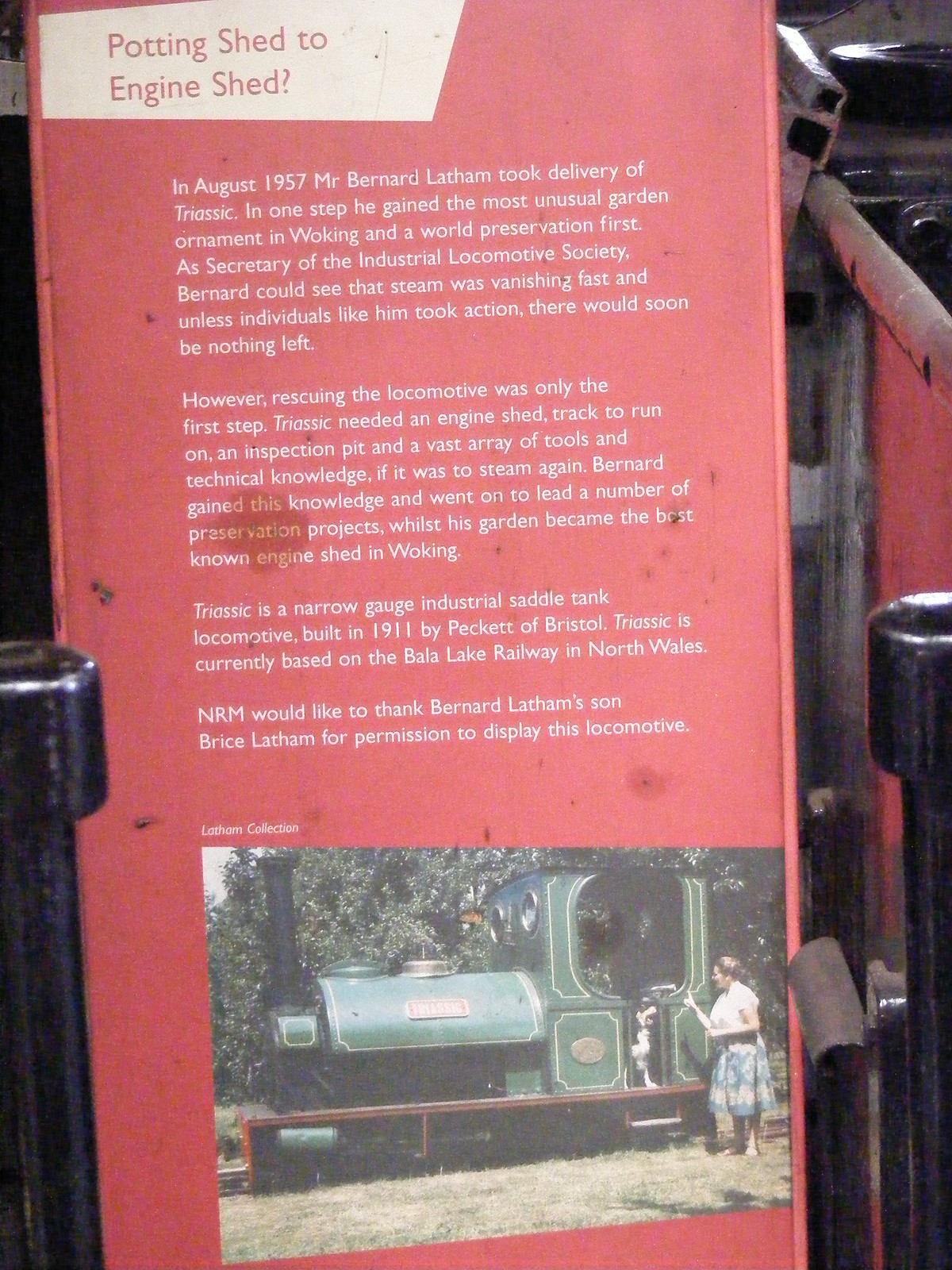This image showcases a red metal plaque with a little white bar at the top left corner, containing the title "Potting Shed to Engine Shed." The text below, all in white, narrates a historical account. It describes how in August 1957, Mr. Bernard Latham acquired 'Triassic,' a narrow gauge industrial saddle tank locomotive built in 1911 by Peckett of Bristol. In one progressive step, he transformed his garden into the most notable engine shed in Woking and achieved a world preservation first. As the secretary of the Industrial Locomotive Society, Bernard recognized the rapid decline of steam engines and undertook efforts to preserve them. Triassic required an engine shed, tracks, inspection pit, and an array of tools to run again, and Bernard's initiatives laid the foundation for several preservation projects. The plaque ends by thanking Bernard Latham's son, Bryce Latham, for allowing the display of Triassic, which is currently based at the Bala Lake Railway in North Wales. Adjacent to this informative plaque is an image of the green locomotive, Triassic, with a woman helping a child near the train, adding a personal touch to the historical narrative.